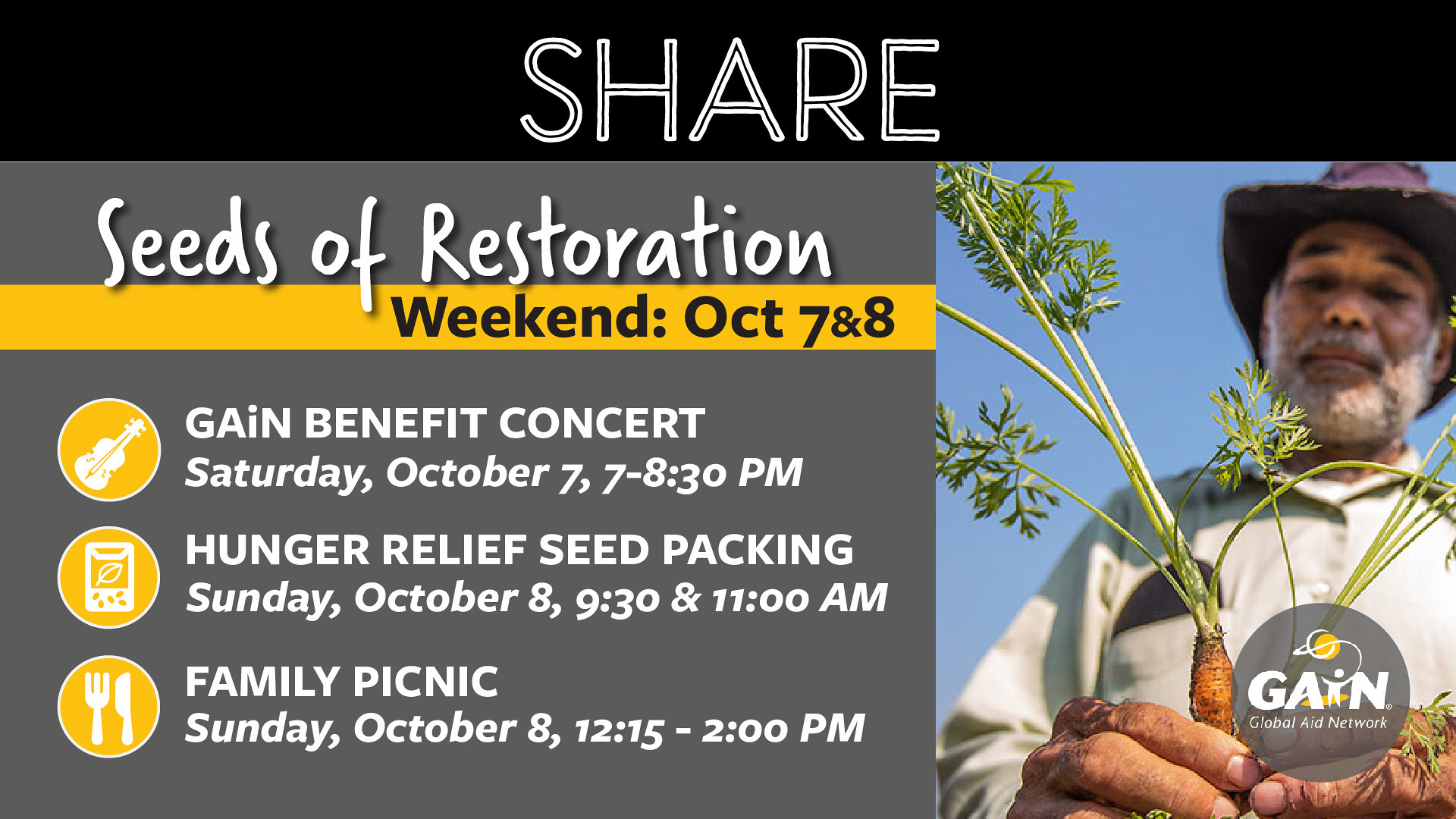The image is a promotional advertisement for an event labeled "Share" prominently on a black bar at the top. Below this, the text "Seeds of Restoration Weekend" is displayed on a gray background with a yellow rectangular highlight. The event spans October 7th through 8th and includes a series of activities listed with corresponding icons on the left. 

- **GAIN Benefit Concert**: Saturday, October 7th, 7:00 p.m. to 8:30 p.m., represented by a yellow circle with a violin icon.
- **Hunger Relief Seed Packing**: Sunday, October 8th, 9:30 a.m. and 11:00 a.m., indicated by a yellow circle with a seed packet icon.
- **Family Picnic**: Sunday, October 8th, 12:15 p.m. to 2:00 p.m., marked by a yellow circle with a fork and knife icon.

On the right side of the image, there is a photograph of a man with a gray beard, wearing a hat and a tan long-sleeve button-up shirt, holding two freshly pulled carrots topped with green leaves and dirt in his hands. The man is associated with GAIN (Global Aid Network), and a logo or label indicating this affiliation is present on his attire. The backdrop of the photograph features a clear blue sky, creating a fresh and vibrant scene.